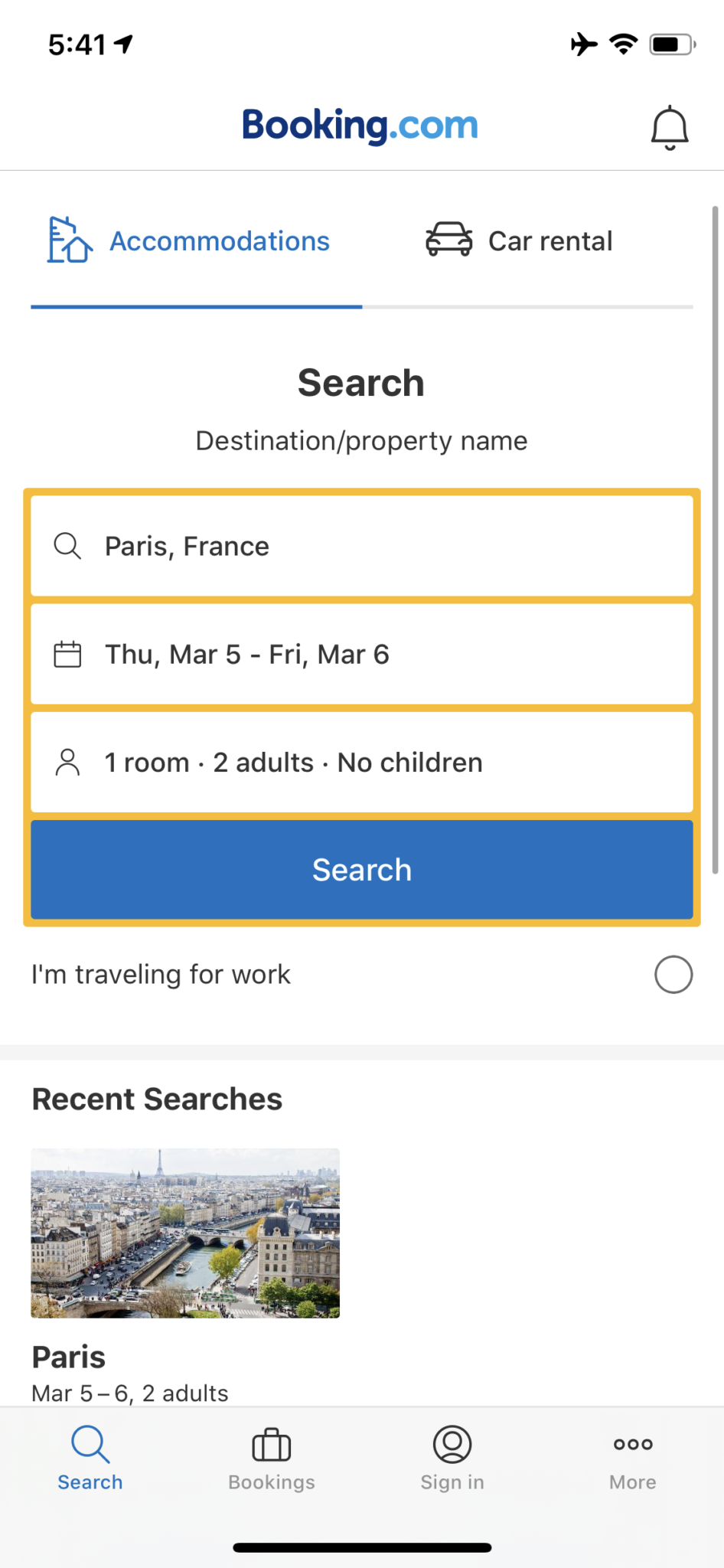The image depicts a user navigating the mobile version of Booking.com on their smartphone. The user is in the process of making a booking for accommodation in Paris, France, specifying a stay for two adults with no children. They are searching for one room from March 5th to March 6th. The screen displays these search parameters prominently, alongside a search button that has evidently been clicked. Beneath this search input, there is a record of a recent search, indicating that the user might have conducted a similar search previously. The screen is organized under a title heading labeled "Accommodation," suggesting that the user is researching possible lodging options in Paris. Additionally, there is a link to car rentals on the right side of the screen, though it remains unselected. The search details reconfirm the intended stay from March 5th to March 6th for two adults, suggesting it is part of the same trip planning process.